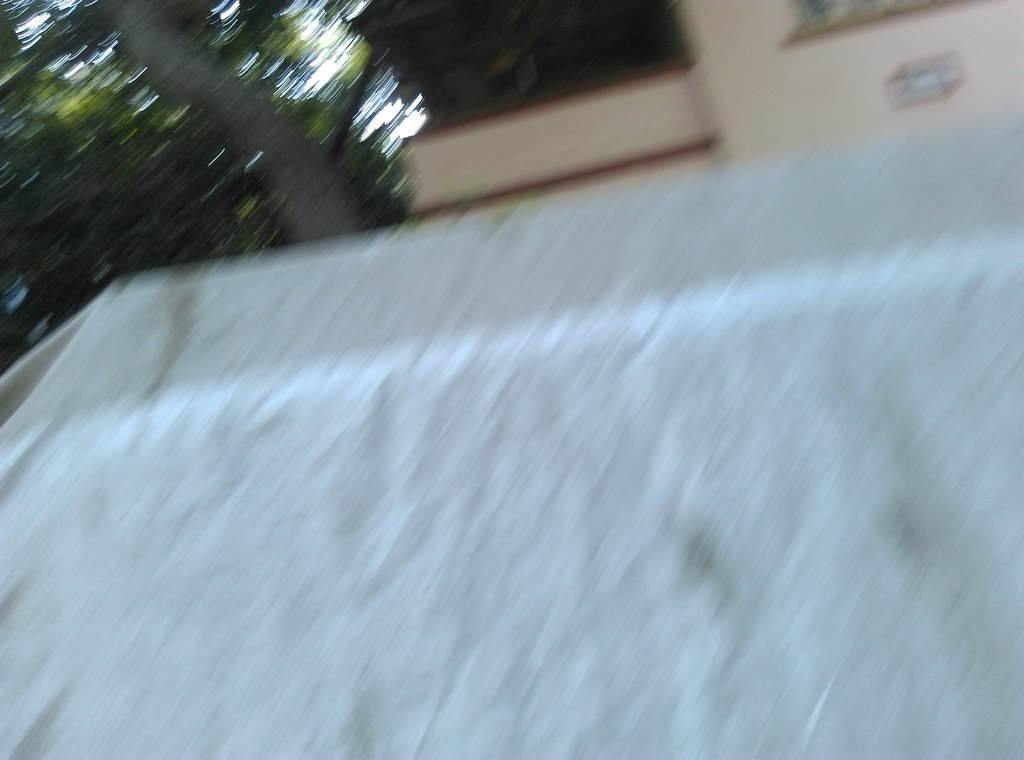This photograph, though blurry, captures a scene from a rooftop amidst ongoing construction. The shot is taken looking upward, offering a partial view of the surroundings. In the upper left corner, a gray tree trunk with abundant green foliage is visible against a patch of sky. The top right features a blonde-colored wooden box with an extension protruding from it. Notably, there is a black outline drawing of a cube on the wooden piece. Dominating the image is a light gray roof that appears to have been recently exposed to wind or rain, as indicated by varied linear markings. The roof's surface also displays contrasting shades of black and is interspersed with bars of light, adding texture to the scene.